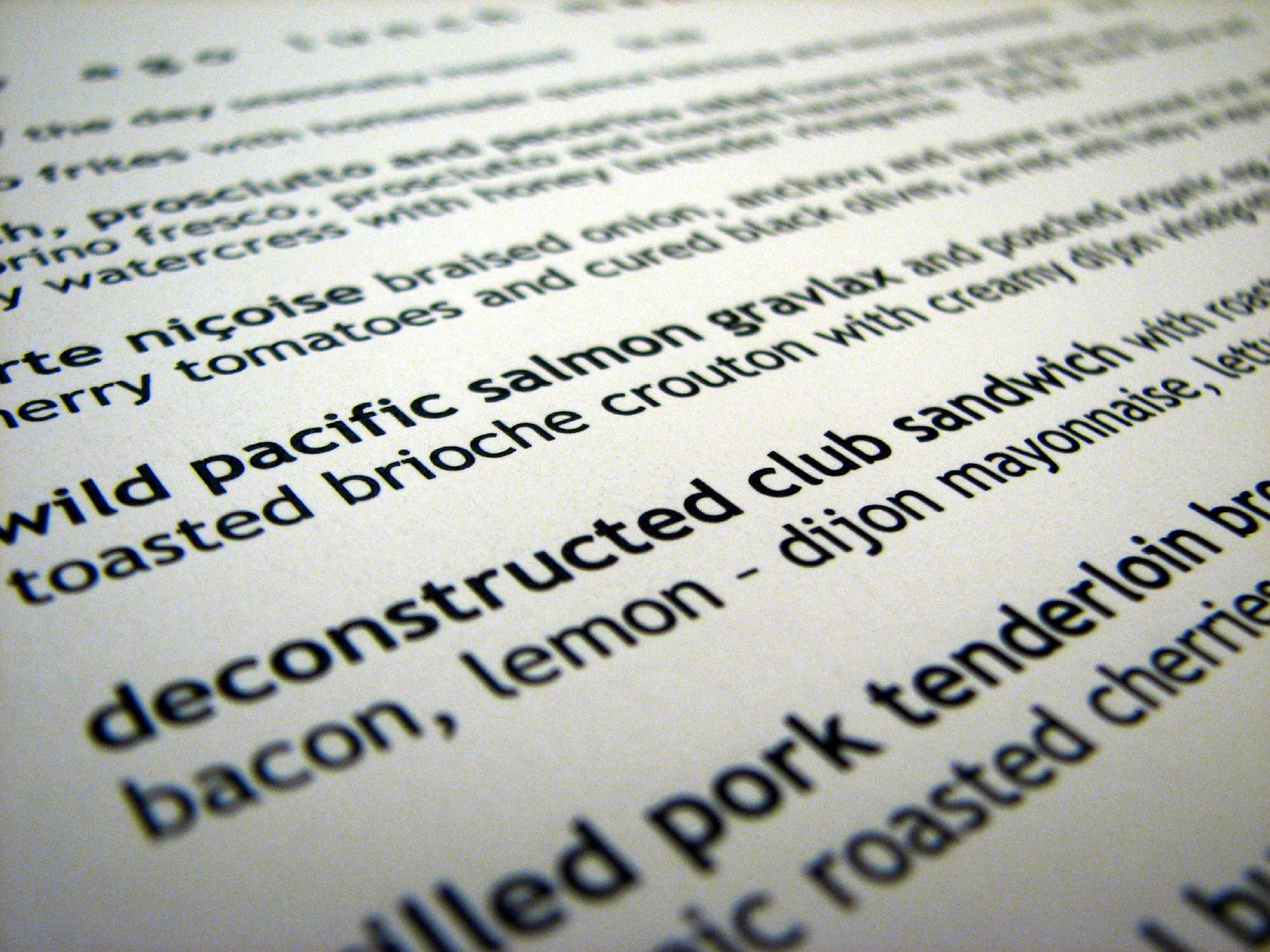The image, captured at an angle, depicts a menu listing for food items taken with a very shallow depth of field, which leaves the foreground and background slightly out of focus. The menu appears on a cream or white background with predominantly lowercase black text. 

In the sharply focused center-left portion of the image, the following food items can be discerned:

1. Nique’s Baked Onion - accompanied by Cherry Tomatoes and Cured Black Olives
2. Wild Pacific Salmon - with Grablax and Poached, continuing with Toasted Brioche Crouton and Creamy Dijon

Moving towards the foreground, the text becomes progressively out of focus, yet parts of the following items remain legible:

- Deconstructed Club Sandwich with Roast, highlighted with Bacon, Lemon, and Dijon Mayonnaise, and partially readable Lettuce
- Pulled Pork Tenderloin and Garlic Roasted Cherries

The overall text tilts diagonally, with the left side lower and the right side higher, enhancing the artistic composition of the photograph. The use of shallow depth of field emphasizes key menu items while fading others into the soft blur of the background.